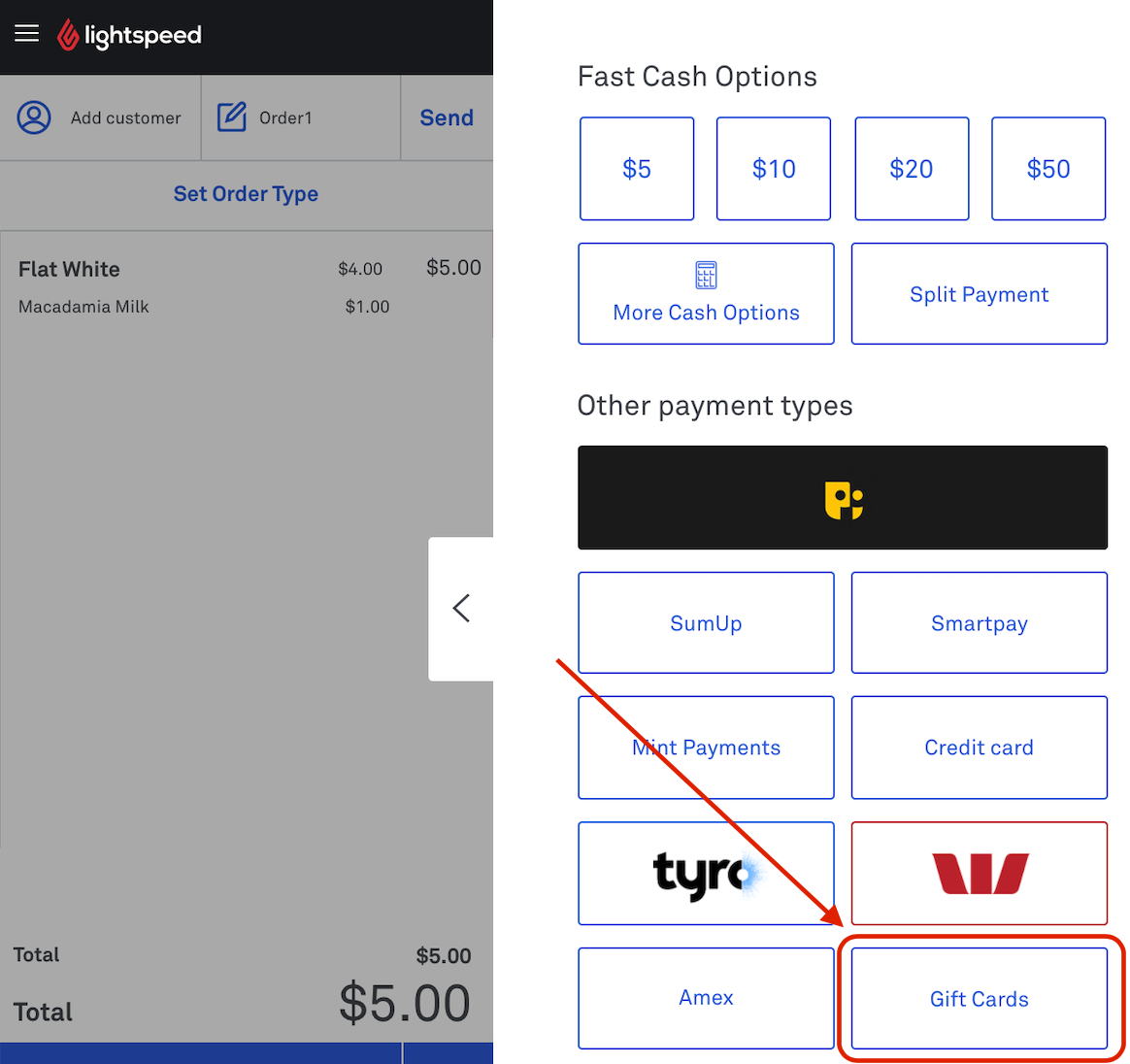The image consists of multiple screenshots within a single frame, predominantly showcasing a point-of-sale system interface. At the top, a black bar prominently displays the label "LightSpeed." Beneath this, set against a grey background, the screen lists several options: "Add Customer" and "Order One." In blue text, it reads "Set Order Type," followed by "Flat White, $4." Notably, the payment is indicated as $5.

Further down, "Macadamia Milk" is listed for an additional $1, bringing the total to $5, as reiterated below with "Total: $5."

To the right, on a white background with blue text and blue-bordered boxes, various payment options are detailed. These include "Fast Cash Options" for $5, $10, $20, and $50. Further options include "More Cash Options" and "Split Payment." Other payment methods such as "SumUp, Smart Pay, Credit Card, Mint Payments, OW, Amex, or Gift Cards" are listed beneath.

A notable detail is that the "Gift Cards" section is encircled by a red line, with a long red arrow pointing to it. This likely indicates that gift cards were the chosen payment method for the flat white with macadamia milk.